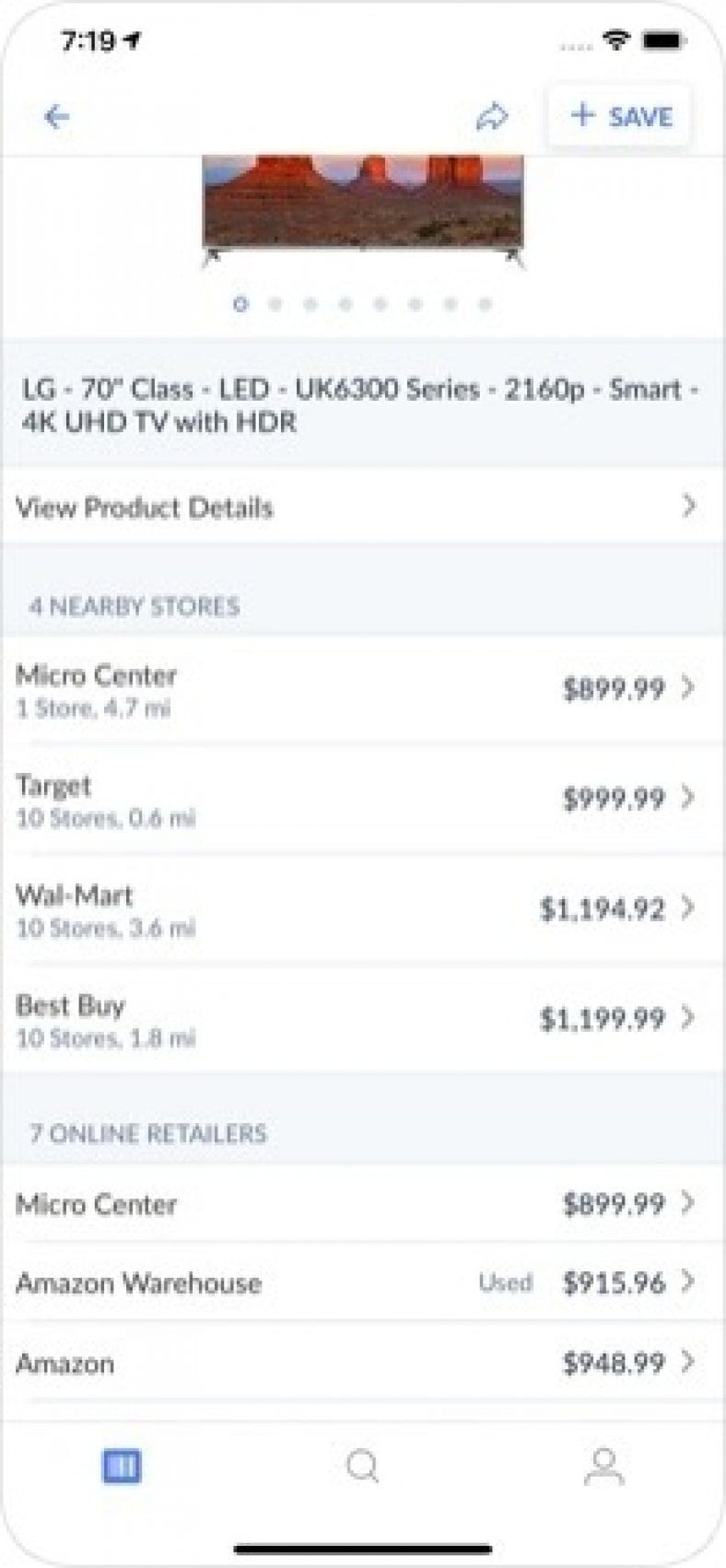This image captures a close-up view of a smartphone screen containing a search result page for a television. The screen displays the time "7:19" in black text at the top left corner, alongside the Wi-Fi and battery icons on the top right. Dominating the upper section, the search result prominently features an LG 70-inch Class LED UK6300 Series 2160p Smart 4K UHD TV with HDR. 

Beneath the image of the partially visible TV, there's a clickable option marked by a right-facing arrow to view the product details. The search results further break down into sections, starting with four nearby stores that have the TV in stock, each listed with prices. Following this, the screen enumerates seven online retailers, detailing their names on the left and corresponding prices on the right, one of which specifies that the TV is used.

The interface includes a blue rectangular or square element at the bottom, whose function is unclear, accompanied by a magnifying glass icon for search and a user profile icon. A black bar marks the central bottom area of the screen, indicating the phone's menu. The predominant background tone is white, interspersed with light gray or blue highlights for specific sections such as "seven online retailers," "four nearby stores," and the TV description.